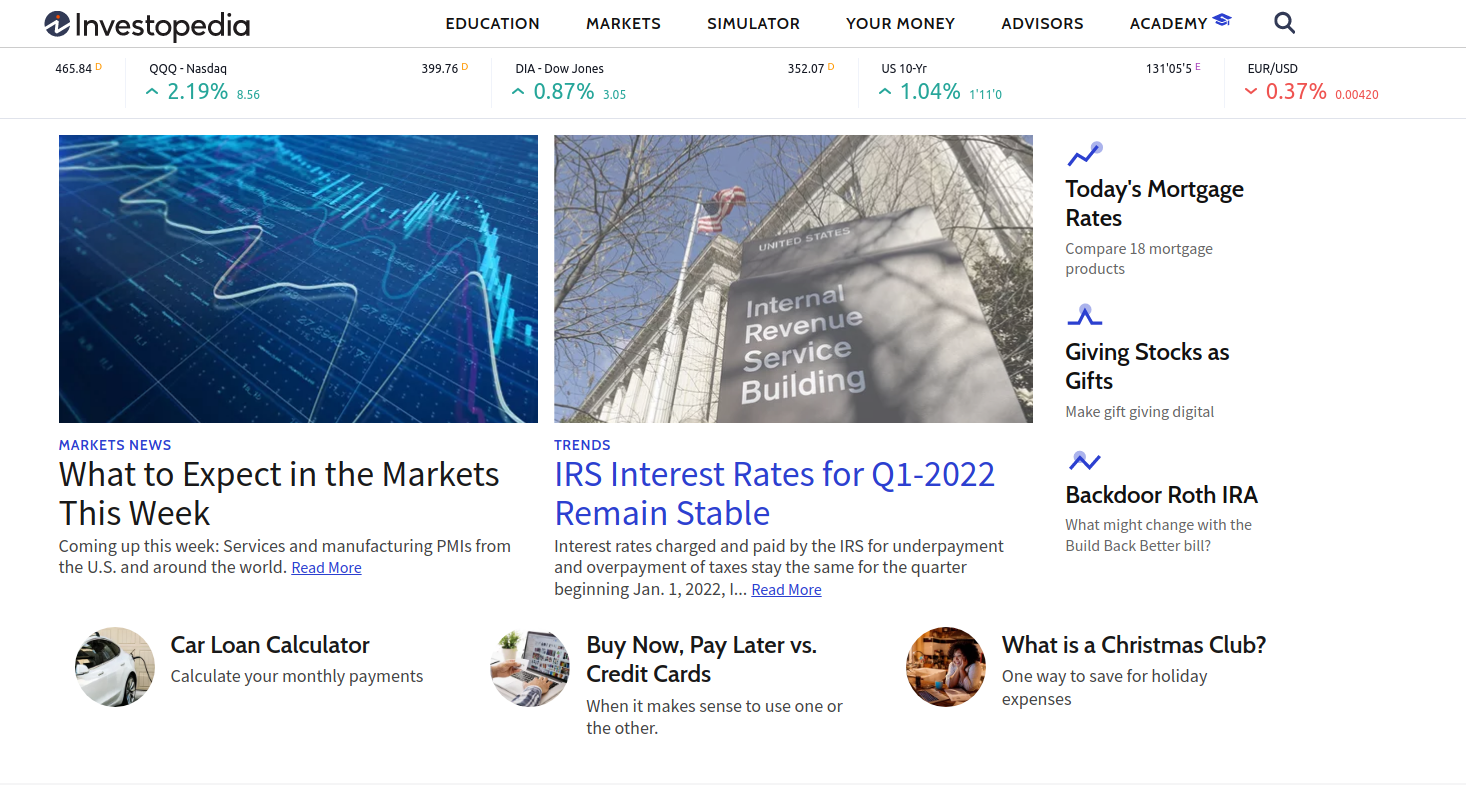The top-left corner of the image displays the Investopedia logo, and to the right, there is a navigation menu featuring options such as Education, Markets, Simulator, Your Money, Advisors, and Academy. Additionally, there is a magnifying glass icon representing the search function. Below the menu, there is a financial summary showing: 

- QQQ-NatDat up 2.19% at 465.84 D.
- DIA-DowJones up 0.87% at 399.76 D.
- US10-YR up 1.04% at 352.07 D.
- Euro to Dollar down 0.37%.

Further down on the left side of the image, a section titled "Market News" highlights upcoming key topics, stating "What to Expect in the Markets This Week," including "Services and Manufacturing PMIs from the US and Around the World" with an option to "Read More." Another section titled "Trends" mentions that the IRS interest rates for Q1 2022 remain stable.